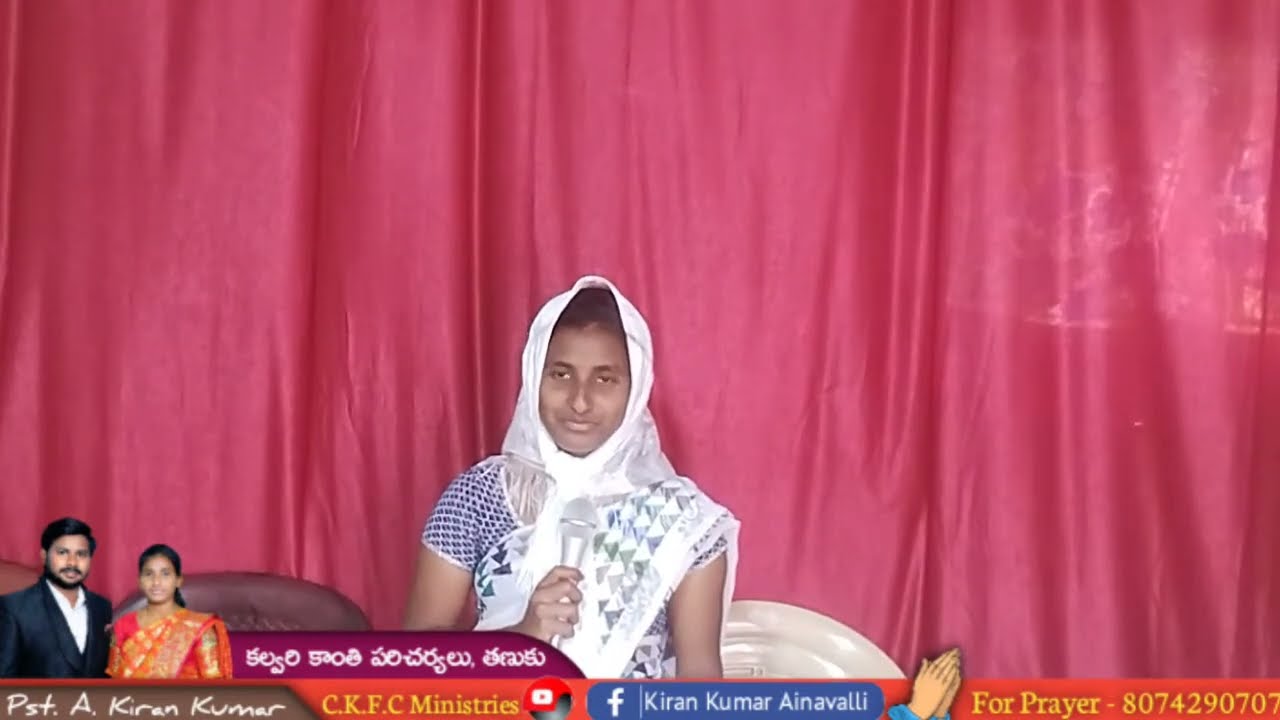The image captures a young Middle Eastern or Indian woman, possibly in her late teens or early 20s, seated slightly to the left of center against a medium red, silky curtain background. The luxurious fabric of the curtain hangs in visible waves and crease lines. The woman is dressed in a blue and white patterned dress and wears a white head covering that drapes over her head, neck, and shoulder. She holds a microphone close to her chin and appears to be on the verge of speaking, projecting a neutral expression.

In the bottom left-hand corner of the image, a man and a woman are visible. The man, dressed in a black suit jacket and white shirt without a tie, stands next to the woman, who is adorned in an elegant red and gold traditional Indian outfit. She, much like the young woman, has a similar cloth draped over her shoulder, but in vibrant red silk.

Below the image content, text elements include "PST A. Kiran Kumar," "CKFC Ministries," a Facebook symbol with the name "Kiran Kumar A. Navali," and an icon of praying hands next to the phrase "For Prayers" followed by the contact number "807-429-0707." This suggests that the setting may be a religious or community event where the young woman is possibly a guest speaker.